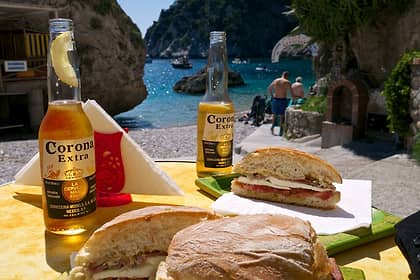This photograph captures a lively outdoor picnic scene set against a picturesque beach backdrop. In the foreground, a table is laden with large sandwiches on sliced rolls, featuring what appears to be white cheese or lunch meat. Alongside the sandwiches are two bottles of Corona Extra, each with different levels of beer remaining—one even adorned with a lime. A red napkin holder with neatly folded triangular napkins adds a touch of casual organization. The background reveals a stunning vista of a crystal-clear, blue ocean bordered by large rocks in shades of brown and gray. To the right, a concrete path with steps leads down to the beach where two white males, one older and one much younger, are walking. The overall scene conveys a sense of enjoyment and leisure, with people interspersing their meal with refreshing dips in the inviting ocean waters.